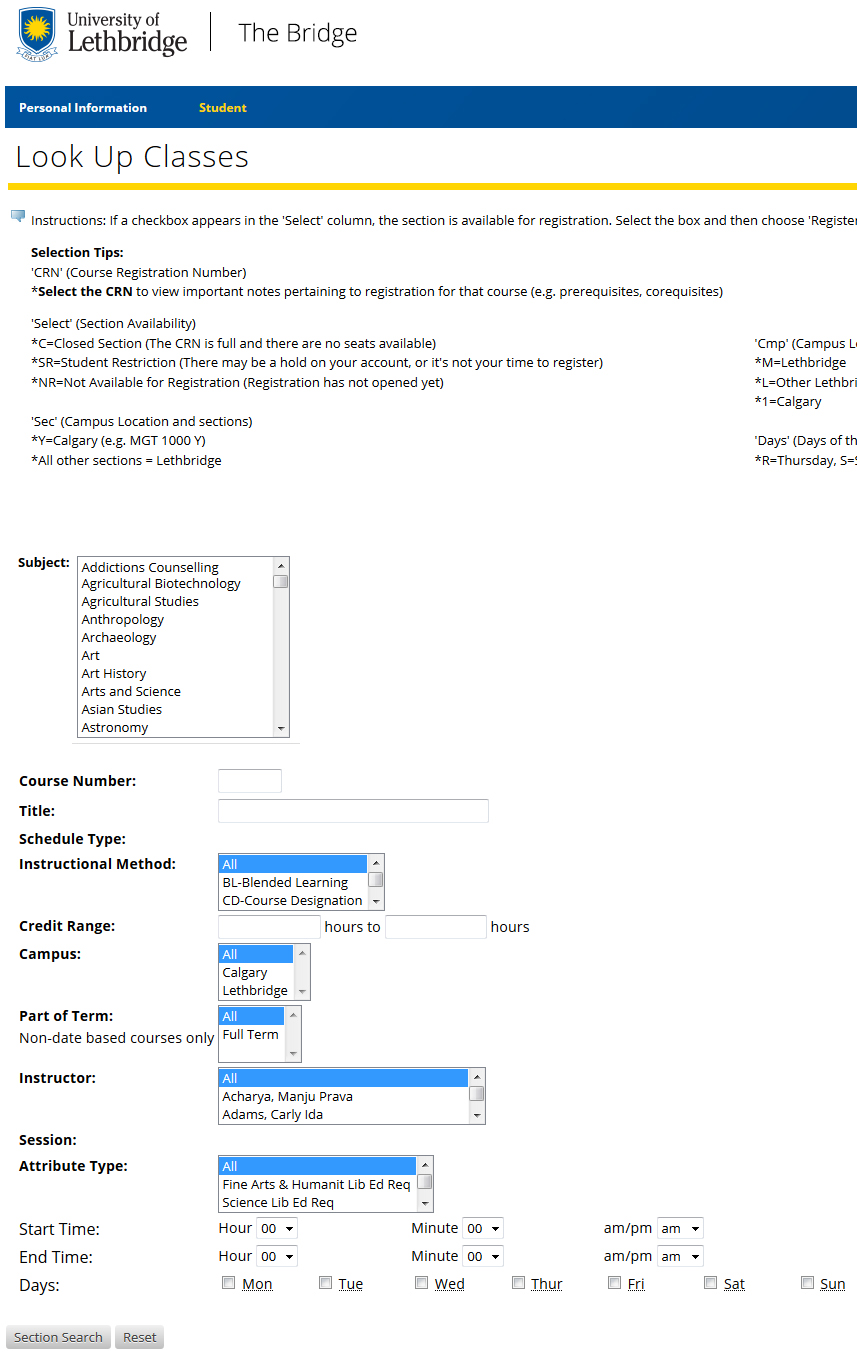This screenshot captures a section of the University of Lethbridge's website, set against a white background. In the upper left corner, "University of Lethbridge" is written in dark gray font, accompanied by the university's seal to its left. The seal is square-shaped with a gold circle at its center, but its small size renders the intricate details and inscriptions indiscernible.

To the right of the university's name, "the bridge" is displayed in light gray font. Below this, a blue header houses the label "Personal Information" in white text, followed by illegible gold text due to its extremely small font size. 

Underneath this blue header, on a white background, the phrase "Look Up Classes" appears in gray font. A yellow horizontal line stretches across the page, marking the beginning of a more detailed section. Below the line, small, unreadable text continues, and further down, the word "Subject" is visible next to a dropdown menu. This menu contains options such as Additions, Counseling, Agriculture, Art, Art History, and Arts and Sciences.

Lower on the page, in black font, labels like "Course Number," "Title," "Schedule Type," and "Instruction Mode" reveal that this is a search form. The form includes multiple search parameters such as Credit Range, Campus, Part of Term, Instructor, Session, Attribute Type, Start Time, End Time, and Days. The fonts used throughout the form are very small, making detailed reading challenging.